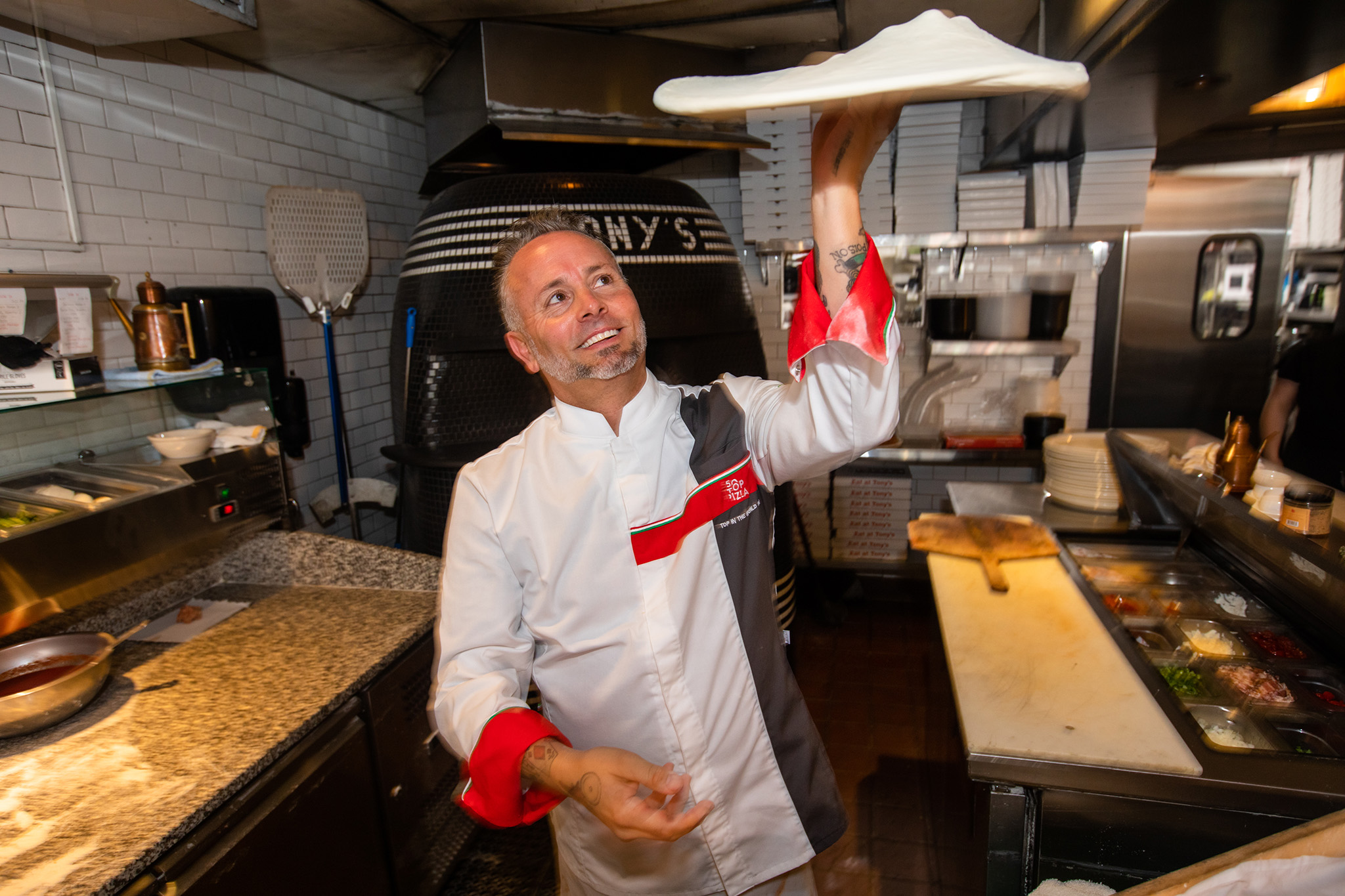In a bustling pizzeria kitchen, a skilled chef, possibly named Tony, is captured mid-action, tossing a disc of pizza dough high into the air. This Caucasian chef, with short gray hair and a neatly trimmed beard along his jawline, is the central focus of the image. He wears a distinctive, button-down chef’s shirt with a high collar that is primarily white, accented with a black stripe down his left side, red cuffs folded back, and a red stripe across his left breast area. His slight smile and upward gaze reflect his concentration as he expertly spins the dough. Behind him, the large, shiny black pizza oven tiled with the letters "O-N-Y-'S" suggests this might be Tony's pizzeria. The kitchen background is a blur of activity, with white-painted brick or tile walls and assorted kitchenware. To his right, a counter is laden with trays of vibrant pizza ingredients—green, yellow, black—while to his left, another counter holds various bowls, napkins, and cooking utensils, adding to the authentic, bustling atmosphere of the pizzeria.